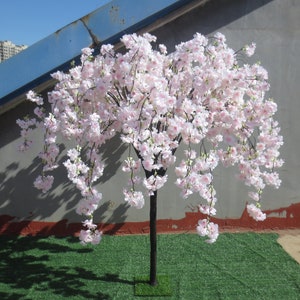This photograph captures a cherry blossom tree in full bloom, situated in what appears to be an urban rooftop garden. The tree, with its slender dark brown trunk, emerges from a patch of vivid, possibly artificial, green grass. The cascading white flowers, tinged with pale pink and centered with deeper pink hues, give the tree a lush and abundant appearance, much like flowing hair. The scene is set against a grey concrete wall, marked by uneven streaks of rust-colored paint at the bottom, stretching up about 10 centimeters. The top left of the image reveals blue skies and multi-storey apartment buildings, suggesting a city environment. A diagonal blue metal beam with rust marks runs across the backdrop, adding an industrial element to this serene botanical display. The cleanliness of the grass and the lack of fallen blossoms indicate the area may have been recently cleaned or maintained, and the tree casts a distinct shadow to the left, hinting at a sunny day. The overall composition of the photograph exudes a contrast between urban elements and natural beauty.